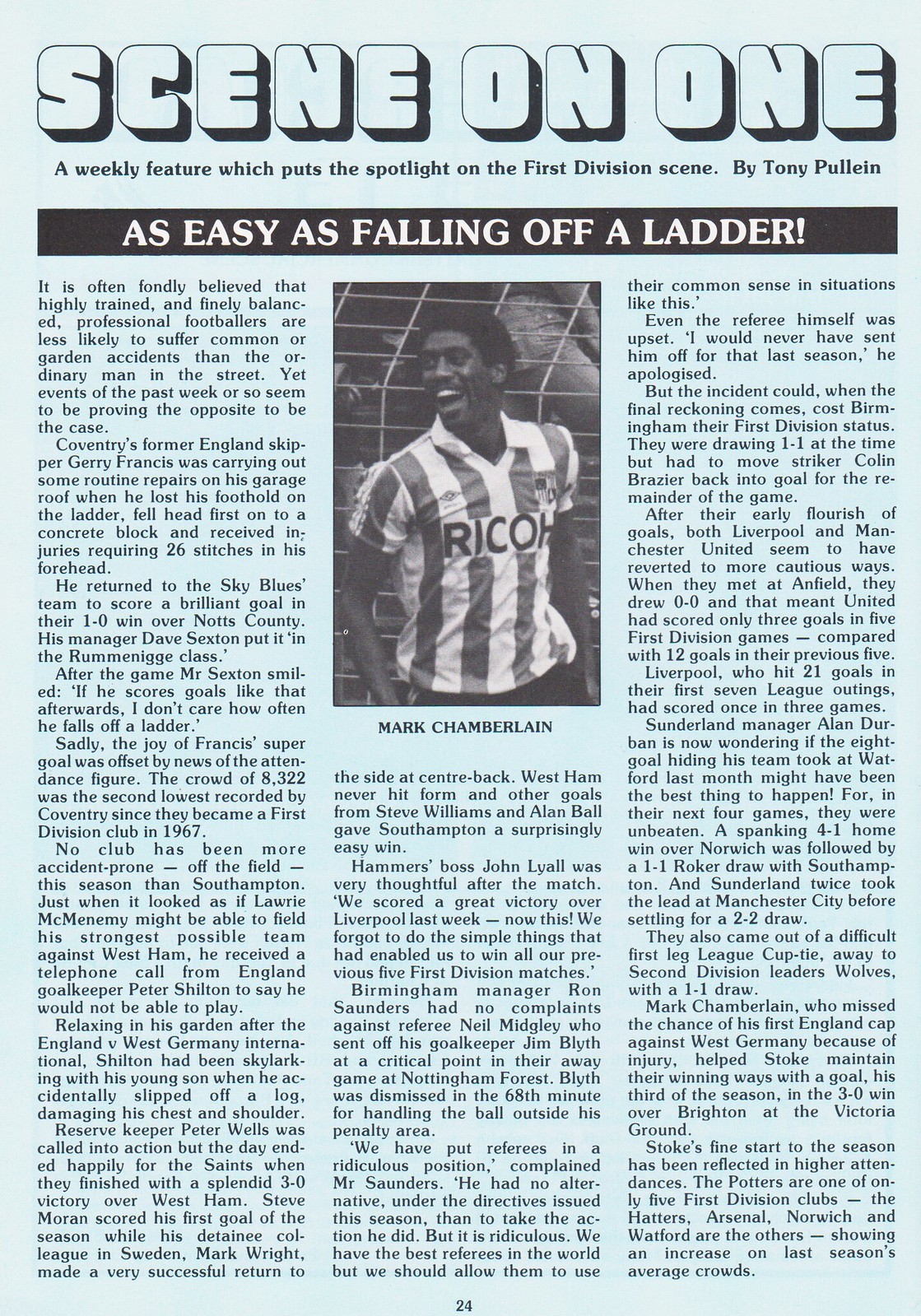This newspaper clipping is from page 24 of a magazine, featuring a light blue background with white bubble letters and a black shadow border at the top that reads "Seen on One: A Weekly Feature Which Puts the Spotlight on the First Division Scene by Tony Poulian." Beneath this heading, separated by a black horizontal bar with white text, is the article titled "As Easy as Falling Off a Ladder." The focus is on a black soccer player named Mark Chamberlain, shown waist-up in the upper middle part of the page, wearing a vertically striped white and gray jersey with "Rico" emblazoned on the front. The article details the story of Coventry's former England captain Jerry Ferraris Francis, who suffered a severe accident while performing routine repairs on his garage roof, resulting in injuries that required 26 stitches to his forehead. Remarkably, he returned to his team, the Sky Blues, and scored a brilliant goal in their 1-0 win over Notts County, an achievement highlighted by manager Dave Sexton. Surrounding the photograph of Chamberlain are three columns of text elaborating on this incident and its implications.